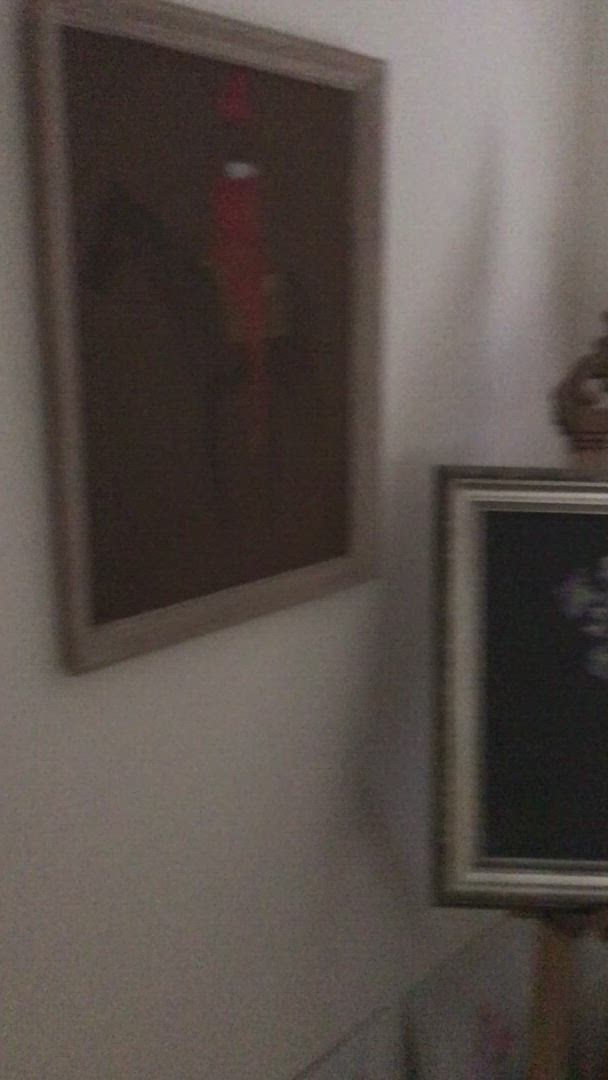The image depicts a white wall with a darker trim at the bottom, which appears to have baby blue wallpaper adorned with floral designs. On the left side of the wall hangs a painting framed in a brass-brown wooden frame. This painting features a man riding a dark brown horse, dressed in a red gambeson and hat, set against a brown background. The frame around this painting is slightly lighter in color compared to the brass-brown frame. Shadows are cast on the wall, adding depth to the scene. To the right of this painting, there is another picture on a dark, ornate easel. This framed picture features a largely black background with a decorative item resembling a snowflake in the upper left corner. The outer brass-brown frame is complemented by a white inner frame. A stand is visible at the bottom right, completing the composition.